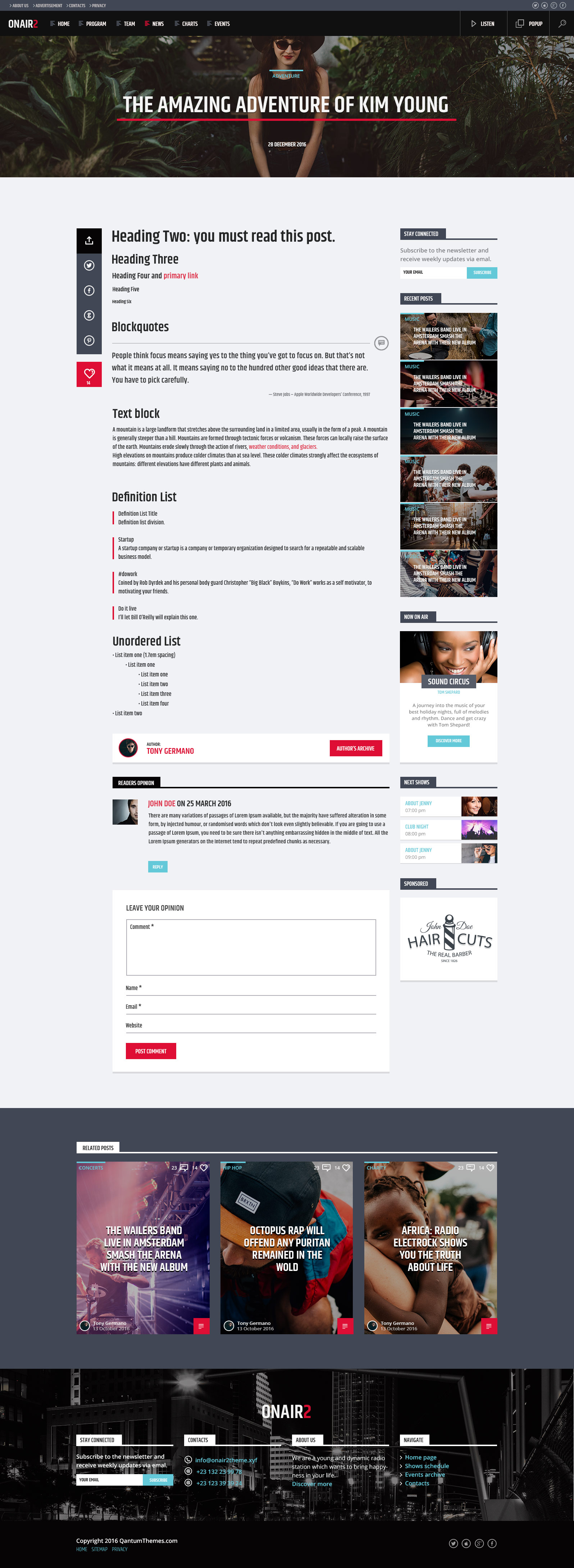The image is a vibrant and detailed webpage layout showcasing an array of content. At the top, the webpage is anchored by a black menu bar featuring navigation options such as 'Home', a login button, and additional links, with a prominent 'On Air' indicator.

Directly below the menu bar is a colorful rectangular header image with a large, bold caption in all capital letters that reads, **"THE AMAZING ADVENTURE OF KIM YOUNG."** This section appears to introduce an article about setting up a website. The focal point of the header image is a middle-aged, Caucasian woman presumed to be Kim Young. She is dressed in a sophisticated black outfit, including a black hat, black shades, and red lipstick, standing amidst a scenic backdrop of trees at sunset. Her arms hang at her sides with her forearms positioned to suggest she is holding her own hands, though her hands are not visible.

Below this main header is an article section with a drop-down menu on the left side. The article section includes a plethora of options such as print, save, and other interactive features. The primary content area starts with a bold prompt, **"You must read this post,"** followed by various typographic elements: headings, block quotes, text blocks, definition lists, and unordered lists, providing a rich, structured layout.

The article is attributed to Tony Jamon. An interactive section below the article allows users to leave their opinions, with an example comment from "John Doe" dated March 25, 2016. There are fields for visitors to input their names, email addresses, websites, and comments.

On the right side of the page, there are links to additional articles, depicted by six thumbnail images with small, indistinguishable captions. Below these thumbnails is an advertisement for "Sound Circus," featuring an African-American woman smiling as she listens to music. This appears to be a clickable promotional banner.

Further down the page, upcoming events are listed, each represented by photos and names of individuals along with event details. 

The final part of the image includes advertisements, most notably for a barber shop, and a section titled "Related Posts" featuring three thumbnails with intriguing captions:
- **"The Realist Man Alive in Amsterdam"**
- **"Octopus Wrap Will Offend Any Puritan Remaining in the World"**
- **"Africa Radio Electric Rock Shows: The Truth About Life"**

At the page bottom, the footer reinforces the title 'On Air', laid over a black background featuring a cityscape with tall buildings and bustling traffic. The footer contains multiple links to different sections of the site, inviting further exploration.

This intricately designed webpage offers a mix of article content, interactive elements, advertisements, and additional multimedia resources, providing a dynamic user experience.